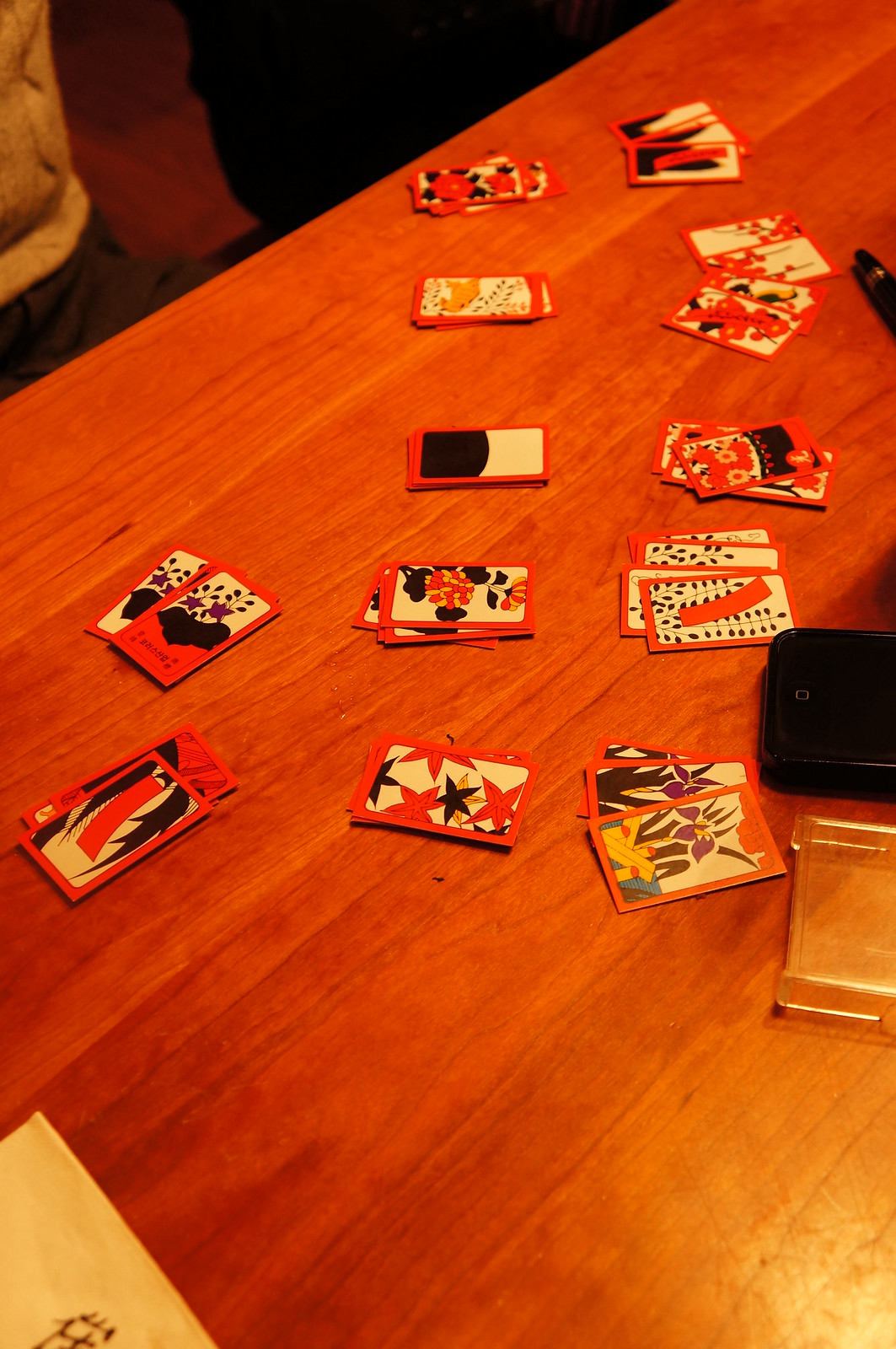The photograph captures an assortment of intricately designed cards scattered across an orangey-blonde wood table. Each card is bordered in orange and showcases various colors and patterns, including black and orange markings, black and orange stars, and blue, green, and yellow hues. Among the designs are several floral patterns, featuring black and purple flowers, black and orange floral motifs, and leaf-like designs in shades of black and orange. Additionally, some cards bear black and white square patterns. 

On the table alongside the cards, the corner of a black smartphone is faintly visible, as well as a black pen lying nearby. To the left of the scene, clothing belonging to two individuals is partially visible—one wearing a combination of white and gray and the other dressed in black. The surface of the table reflects light, adding a gentle sheen to the scene. A white sheet of paper adorned with graphics lies amongst the items, and a clear square object is also present, contributing to the array of elements in the photograph.